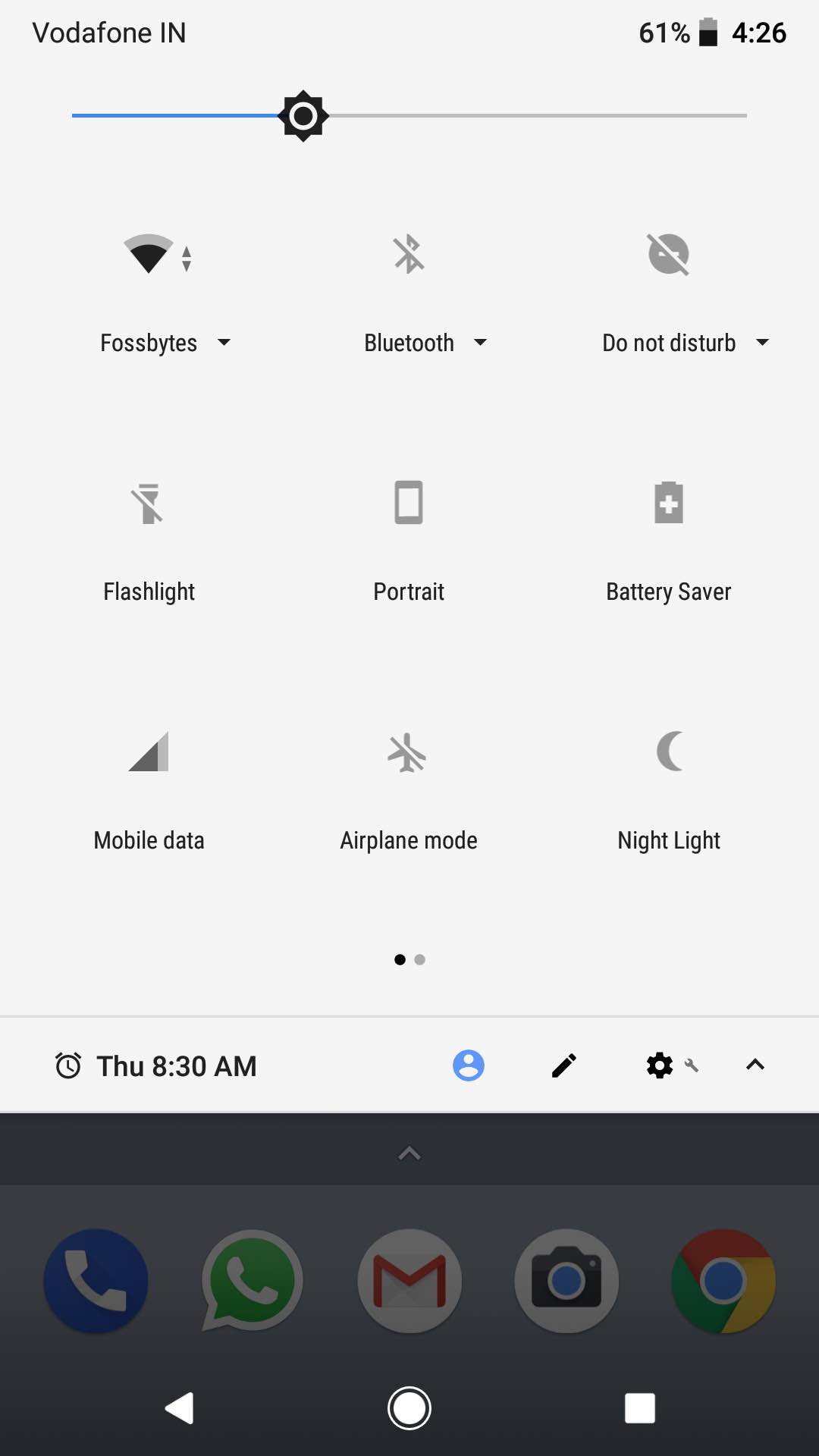This screenshot from a mobile phone display features a light gray background. In the upper left corner, "Vodafone IN" is displayed in black text, while the upper right corner shows a battery icon at 61% and the time "4:26." Directly beneath this is a status bar, approximately one-third blue, with a gear icon on the right end, followed by a gray remainder.

Below this, arranged into three rows of icons and labels:

- The first row includes:
  - A fan icon with the label "Phosphites."
  - A Bluetooth icon with a slash through it and the label "Bluetooth."
  - A Do Not Disturb icon with the label "Do Not Disturb."

- The second row contains:
  - A flashlight icon with a slash and the label "Flashlight."
  - A phone icon with the label "Portrait."
  - A battery icon with a plus sign and the label "Battery Saver."

- The third row features:
  - A triangle icon labeled "Mobile Data."
  - An airplane icon with a slash through it and the label "Airplane Mode."
  - A moon icon labeled "Nightlight."

Adjacent to these icons are three dots in black, gray, and white, aligned above a thin gray line. Below this section, an alarm clock icon is displayed with "THU 8:30 AM." 

Towards the bottom, several icons are lined up, including:
  - A people icon.
  - An edit icon.
  - A settings icon.

The lower portion of the screen, slightly grayed out, features five distinct app icons: 
  - A phone app.
  - WhatsApp.
  - A mail app.
  - A camera app.
  - The Chrome browser app.